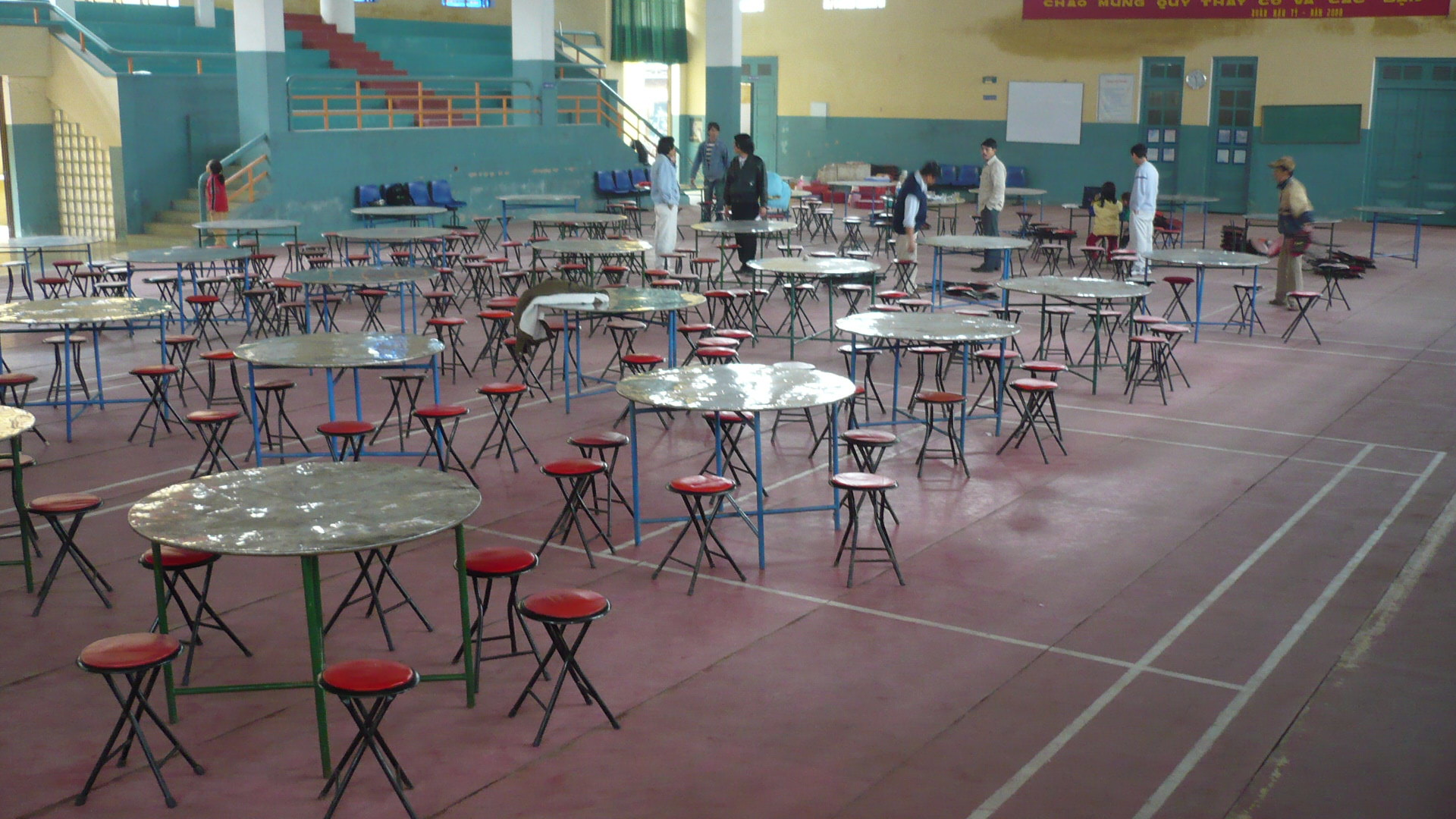The image depicts an expansive cafeteria room filled with circular metal tables featuring shiny silver tops. Each table is supported by colorful pipes in either green or blue and surrounded by five or six stools without backrests. These stools have black legs and circular cushions, some described as "little red stools with black legs that appear to fold up." The floor is composed of large, light red or pink stone rectangles. In the background, towards the top left of the photo, a large blue staircase with yellow accents leads to an auditorium-like seating area. Scattered around the room, a few people in various colored outfits can be seen conversing, adding life to the scene.